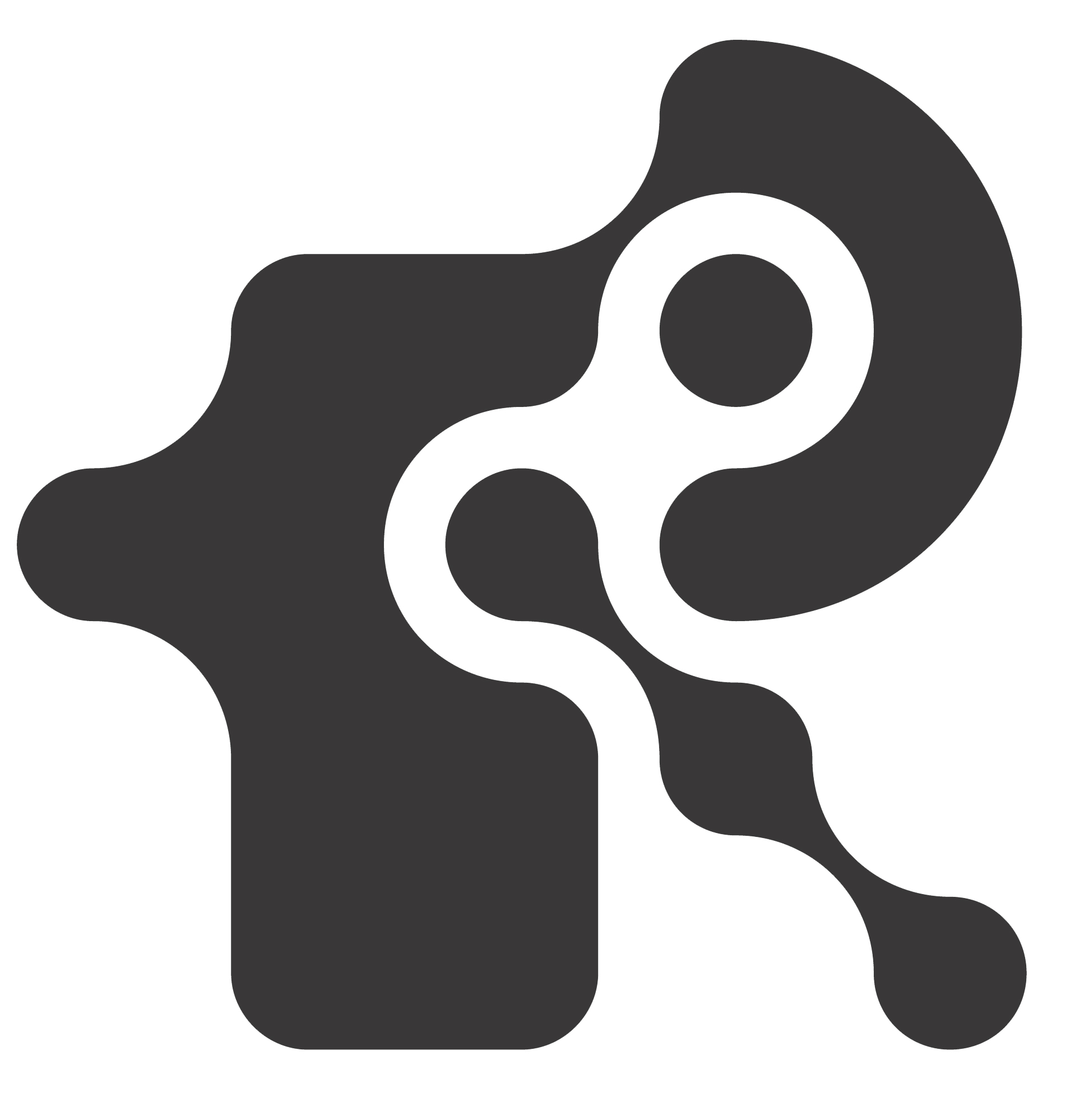The image showcases a striking abstract composition on a plain white background, featuring a harmonious interplay of three black shapes, all in the same shade of black with smooth, rounded corners and curves that create a bubbly, circular appearance. 

The most prominent shape begins in the bottom left-hand corner, ascending towards the top left and sweeping across the top right in a backwards C formation. Encased within the curve of this backwards C is a central black circle, adding a focal point to the fluid design.

Intersecting this larger shape from the bottom right side of the image, a unique form resembles a straight line with bulbous, circular protrusions, disrupting part of the larger black shape and positioning itself roughly in the middle of the composition. This amalgamation of shapes creates a dynamic visual contrast against the stark white backdrop, melding fluid motion with abstract geometric precision.